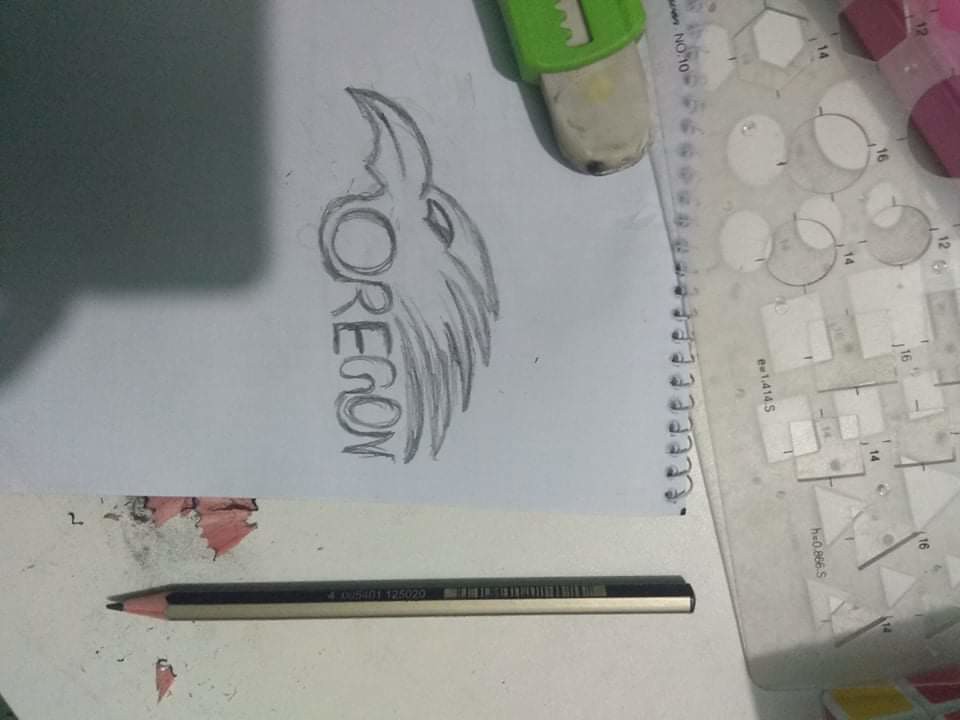This image features a detailed pencil drawing on a sheet of paper that is oriented sideways. At the top of the paper is an eraser, and to the right lies a stencil containing various shapes, including circles, octagons, and triangles. At the bottom of the image, a gold-colored, freshly sharpened pencil is placed, accompanied by its shavings. 

The notebook itself, or possibly just the perspective of the image, is sideways. The word "Oregon" is inscribed in pencil, with the "O" artistically integrated into a design resembling a bird's head. This bird head, reminiscent of an eagle, is characterized by a pointed, slightly rounded beak, and feather-like patterns at the rear of the head. A shadow casts over the paper, adding depth to the scene. Beneath the stencil, there appears to be a pink pencil case or possibly a box, partially visible.